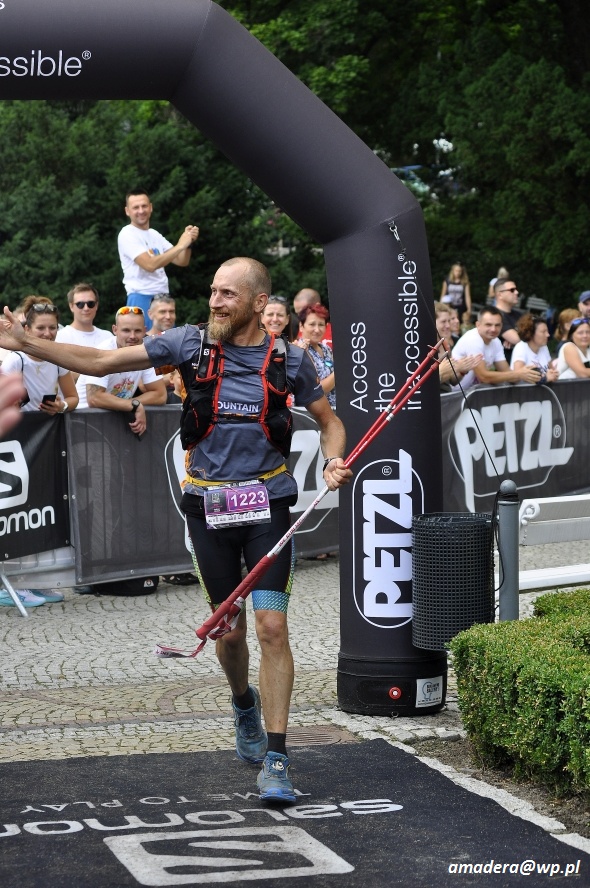In this outdoor photograph, a bearded man, approximately 45 years old, is captured mid-stride, participating in what appears to be a sporting event. He is dressed in athletic attire, comprising black running shorts with a blue trim, a dark gray shirt emblazoned with the word “Mountain,” and a small black vest accented with red piping. A watch adorns his arm, and he's equipped with two red poles, which he holds in one hand, suggesting a specialized sporting activity.

The man exhibits a cheerful demeanor, smiling and waving toward the crowd as he runs underneath an inflated arch. This arch marks the passage over a gray mat inscribed with the upside-down logo "Salomon Time to Play." His feet are shod in blue running shoes complemented by black socks.

The background reveals a modest crowd of approximately 20 spectators, stationed behind a black-and-white advertising barrier promoting "Petzl." Some among them are smiling and applauding, with one person notably clapping. A trash can is visible to the right of the scene, positioned near some green, densely leafed bushes that frame the spectators, adding a touch of nature to the event's setting.